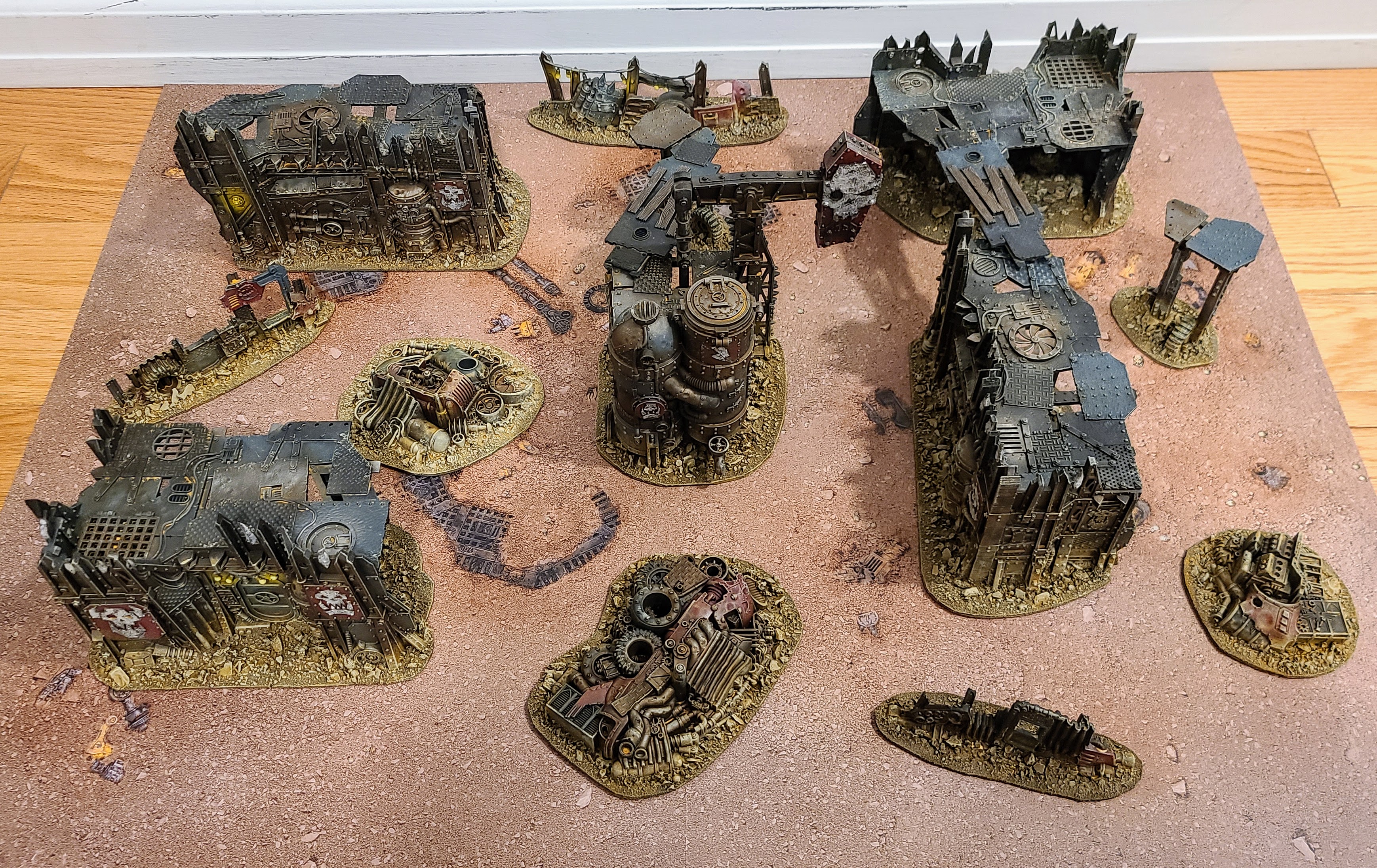This is a highly detailed, full-color indoor photograph of a curated tabletop display, likely designed for a dystopian or steampunk-themed role-playing game. The square image, staged using artificial lighting, features an array of intricate miniatures set against a backdrop of a light brown hardwood floor and a white baseboard. 

The center of the composition is dominated by an orange-brown metallic platform supporting numerous dark, industrial-looking models. In the bottom left corner, there's a striking castle with two prominent towers. Adjacent and central, a large mansion with cylindrical turrets evokes an old, factory-like aesthetic, complete with a wheel in the background. A series of flat-roofed buildings extends across the scene, connected by planked walkways; one such building resembles a church with a spire and columns.

Other notable elements include bases showcasing a variety of small buildings and objects, such as cogs, exhaust pipes, and possibly scrapped vehicles, reinforcing the dystopian theme. Pillars, intricate metalwork, and even a solitary door with a window add to the complexity of the arrangement. Multiple pieces are adorned with clockwork, metal pieces, and skull emblems, enhancing the dark, spooky, and industrial ambiance. This visually rich display is positioned on a staged terrain, meticulously blending with the overall setting.